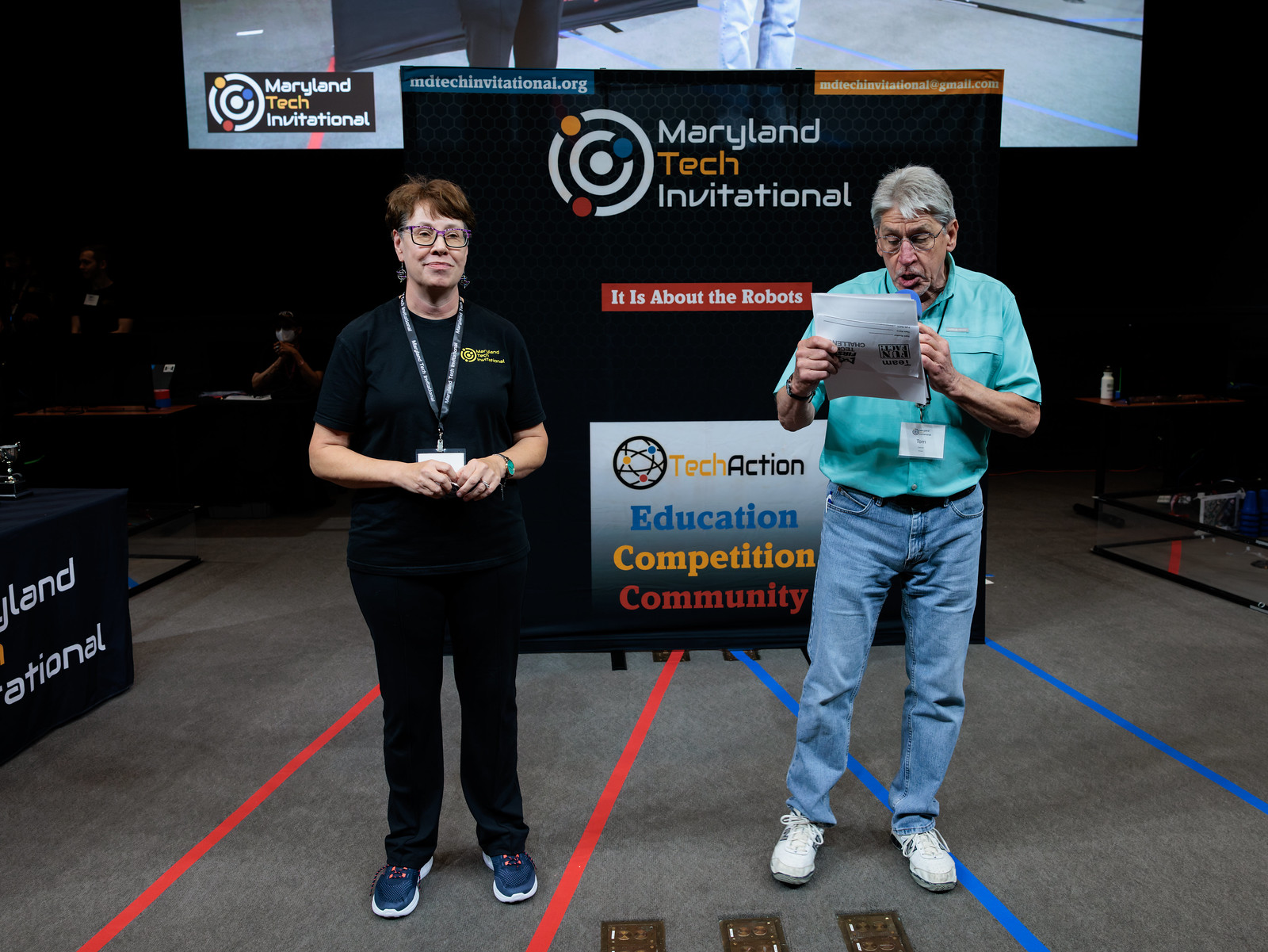In this detailed image, we see a man and a woman standing in front of a towering advertisement board—approximately 10 feet tall—that reads "Maryland Tech Invitational" along with "Tech Action, Education, Competition, Community" at the bottom. The vibrant logo on the board features a red target circle filled with yellow, blue, red, and white highlights. The woman, standing to the left, has short brown hair and wears glasses. She is dressed in a black t-shirt and black pants, complemented by blue athletic shoes with orange shoelaces, and she has a lanyard around her neck, hands folded in front of her. The man beside her, holding a blue microphone and reading from a piece of paper, wears a light blue short-sleeve shirt, blue jeans, and white sneakers. He also has short gray hair and a lanyard around his neck. The background includes tables with a few people seated, indicating the indoor setting with gray carpet. This lively scene is set at a robot-centric event in Maryland, hinting at a dynamic and engaging atmosphere.